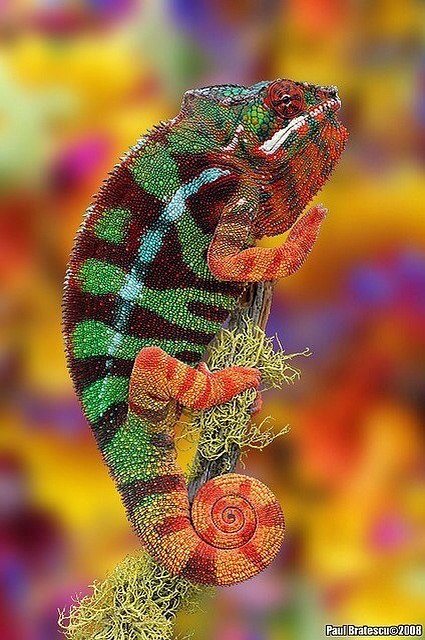This vibrant photograph, set in portrait orientation, features a colorful chameleon perched on a green, fuzzy twig, set against an abstract, psychedelic background that swirls with hues of yellow, blue, orange, red, pink, and purple, giving a dreamlike effect reminiscent of flowers. The chameleon’s body is an intricate display of diverse colors, primarily green and dark red, with striking patterns. Its legs and tail exhibit vivid orange, red, and yellow stripes, with the tail elegantly curled into a spiral. The chameleon’s head, showcasing a small eye and nose, is adorned with little spikes along its back and boasts a distinctive hanging throat flap that is red with green stripes. The mouth is defined by a white line. The image, created by Paul Bradescu in 2008, captures the essence of photographic realism, blending lifelike detail with a surreal background.